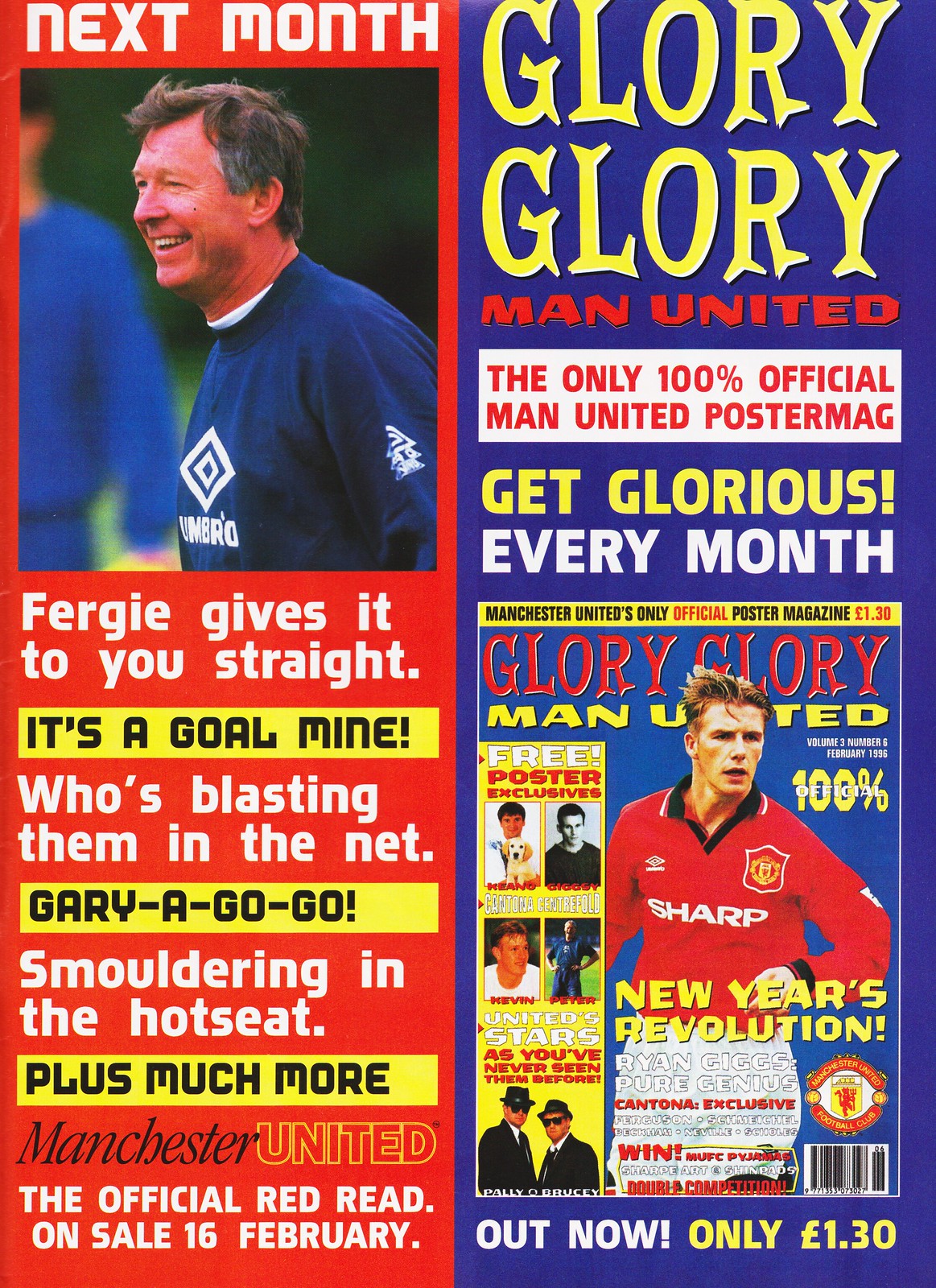The image is a rectangular cover page of a magazine or program, predominantly featuring red on the left side and blue on the right. At the top left, the text "Next Month" is printed in white, followed by a photograph of a man clad in a blue jersey with the Umbro logo prominently displayed. Beneath the photo, several headlines are listed: "Fergie Gives It to You Straight," "It's a Gold Mine," "Who's Blasting Them in the Net?" and "Gary A-Go-Go, Smoldering in the Hot Seat, Plus Much More." The section wraps up with "Manchester United: The Official Red Read, On Sale 16th February."

On the right side, the text "Glory Glory, Man United, the Only 100% Official Man United Poster Mag" stands out, accompanied by "Get Glorious Every Month." This part also features the cover of another issue of the magazine, showing a player in a red jersey and white shorts, indicative of more detailed content about Manchester United. The bottom of the image concludes with the announcement, "Out Now Only 130e," highlighting the magazine's availability and price. 

Overall, the cover combines striking colors and dynamic text to promote exclusive insights and content related to Manchester United.